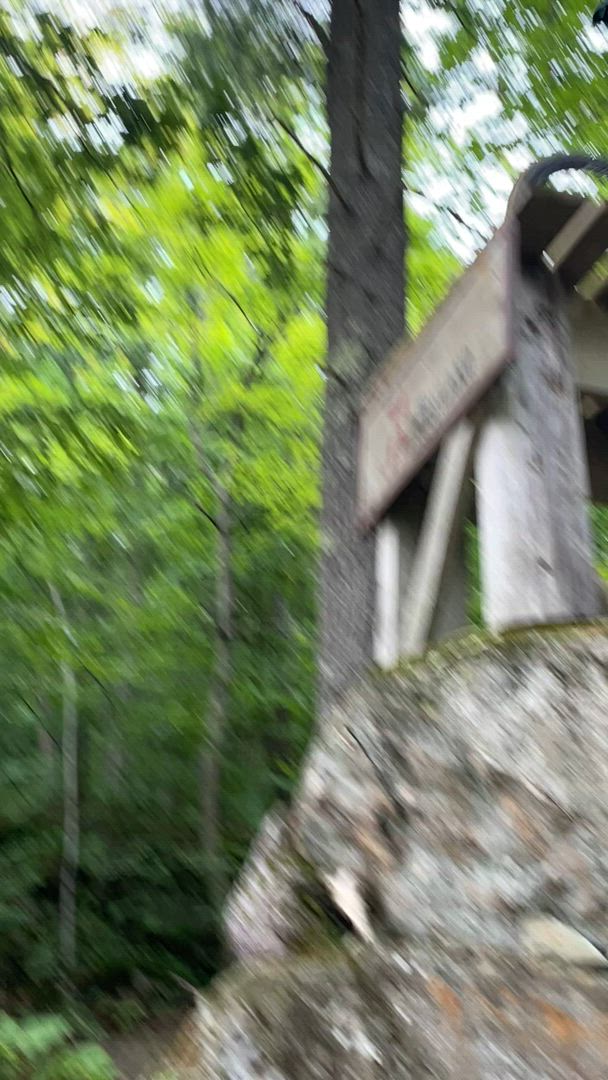This photograph, taken outdoors, captures the vibrant scenery of what appears to be a park or trail, although the image is quite blurry, suggesting the photographer was in motion. In the background, there is an abundant grove of bright green leafy trees that seem to be young, given their relatively short height and thin trunks. The trees are densely covered in fresh, healthy foliage, which, along with the vivid green hue, indicates that the season is likely spring or summer. In the bottom right corner of the image, there is a rocky outcrop adorned with a wooden structure featuring a rounded roof. Despite the blurriness, the structure seems to have a sign on it, although the details of the sign remain indistinguishable.